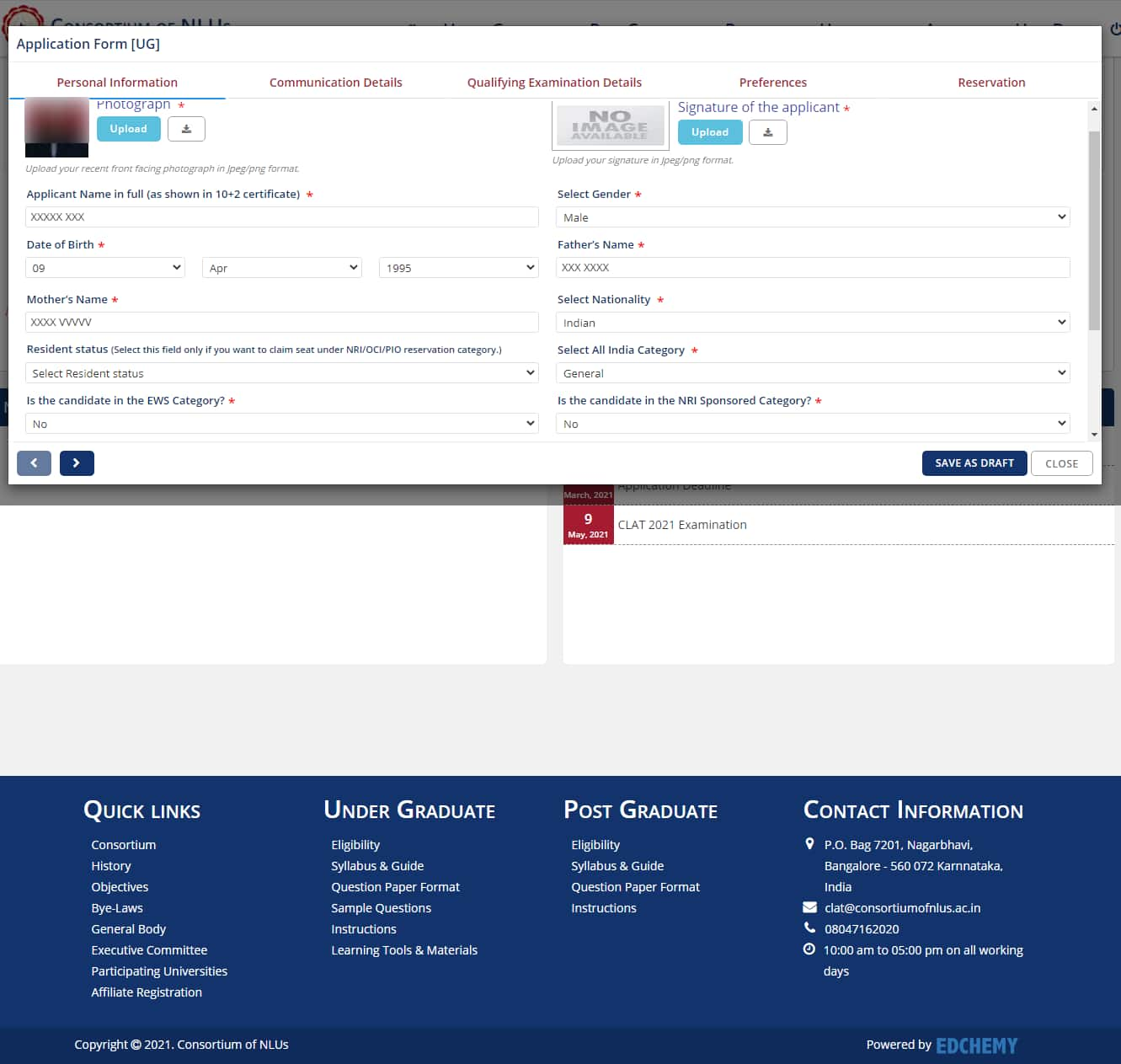The screenshot features a website displaying an application form, predominantly white with a navy blue bottom section that contains white text. In the bottom right-hand corner, the text "Powered by EdChemE" is visible. The application form is presented as a pop-up where users can input their personal information, communication details, qualifying examination details, preferences, and reservation status. 

Currently, the "Personal Information" section is selected. This segment allows applicants to upload a photograph and a signature, each facilitated by baby blue upload buttons positioned on the left and right sides, respectively. Below the photograph upload section, there are fields for the applicant's full name, date of birth, mother's name, resident status, and EWS category status. 

On the right side, beneath the signature upload section, applicants can select their gender, provide their father's name, confirm their nationality, indicate their All India category, and specify if they are in the NRI sponsored category. 

At the bottom of the form, options exist to switch to the "Communication Details" page, save the application as a draft, or close the form. Behind the pop-up application form, the date "May 9, 2021" for the CLAT 2021 examination is visible. Furthermore, the bottom section of the screenshot contains quick links under the "Postgraduate" section and contact information.